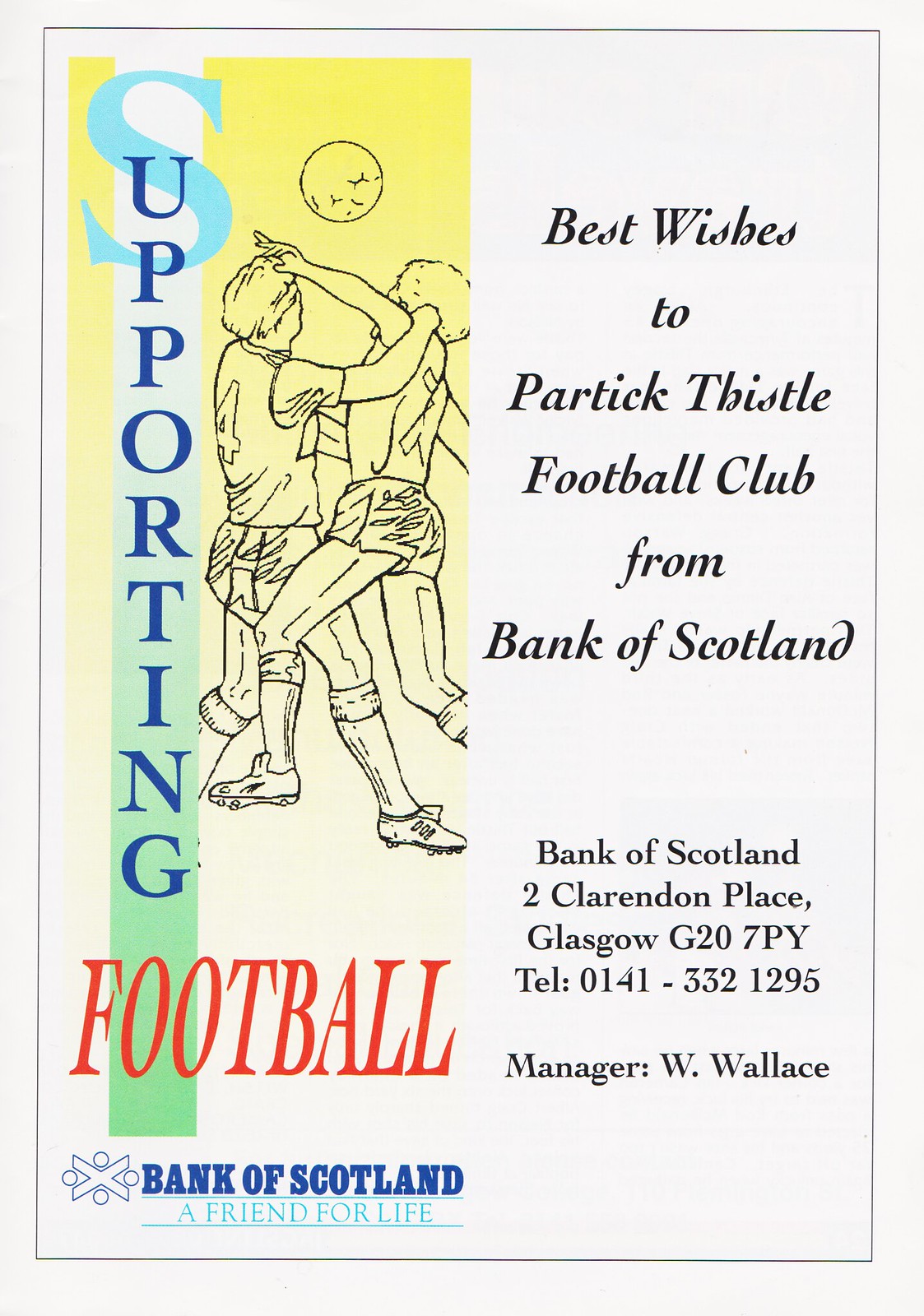This is a detailed advertisement supporting the Partick Thistle Football Club, created by the Bank of Scotland. The flyer prominently features a rough sketch on the left of two soccer players fighting over a ball in the air, seemingly colliding. The text is colorful, with "Supporting Football" written vertically in blue and red beside the drawing. To the right, the message "Best wishes to Partick Thistle Football Club from Bank of Scotland" is clearly stated. Another line below declares, "Bank of Scotland, a friend for life." The advertisement also includes contact details: Bank of Scotland, 2 Clarendon Place, Glasgow, G20 7PY, Telephone 0141-332-1295. The manager, W. Wallace, is also mentioned, indicating the bank’s support and connection to the club.